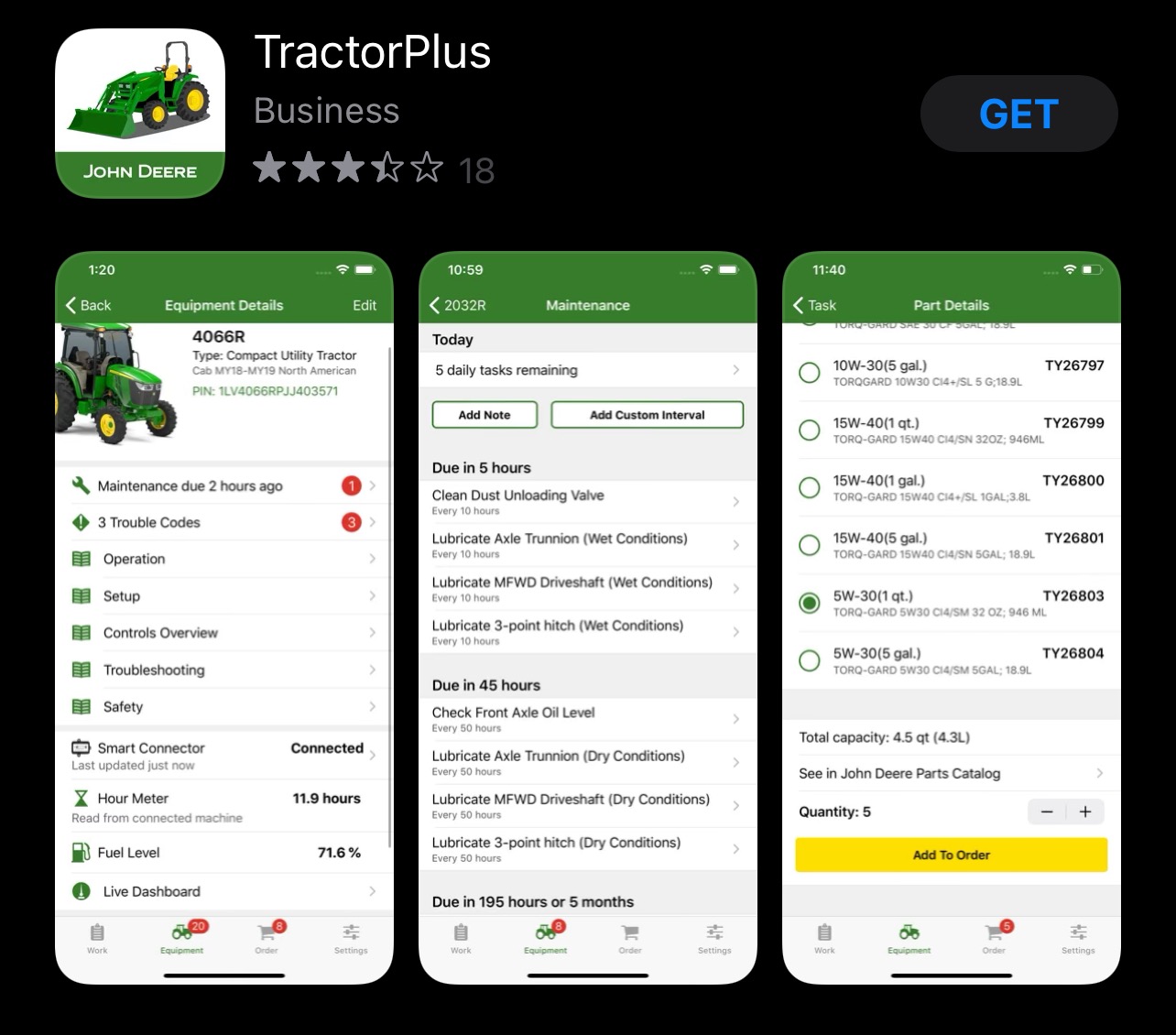In the image, we see the Trexel Plus Business app displayed on the Apple Play Store, accessible via the Apple Store. The app has been rated 3.5 stars by 18 users, with the stars and rating both shown in grey, while the unrated stars are black. The top left corner of the image features the app name "Trexel Plus Business" written in white and grey against a black background. To the right, there is a blue button with a black background labeled "cat." Adjacent to the app name on the left is an icon depicting a green Trexel with yellow rims and black tiles, set against a green board.

Below this, "John Dee" is displayed alongside three screenshots of the app's interface on a smartphone. The leftmost screenshot shows equipment details, highlighting a green John Deere tractor with essential information like maintenance due hours, trouble codes, operational setup, control over fuel, troubleshooting, safety measures, smart connect status, hour meter (9 hours), and fuel level (71%). It also features a live dashboard.

The central screenshot focuses on maintenance tasks for the day, listing five remaining tasks, including cleaning dust valves, lubricating axles, trunnions, oil condition checks, and specific intervals (2 and 5 hours) for various lubrication tasks.

The rightmost screenshot provides parts details, with the selected part labeled "5WDD." It notes the total capacity (4.5 quarts or 4.3 liters) for the engine, a parts catalog with five items, and an "air to water" button highlighted in yellow. Below, functionality buttons for work equipment, order, and settings are present. The maintenance section at the top is green, while the main interface has a white background with black text and green icons on the left side.